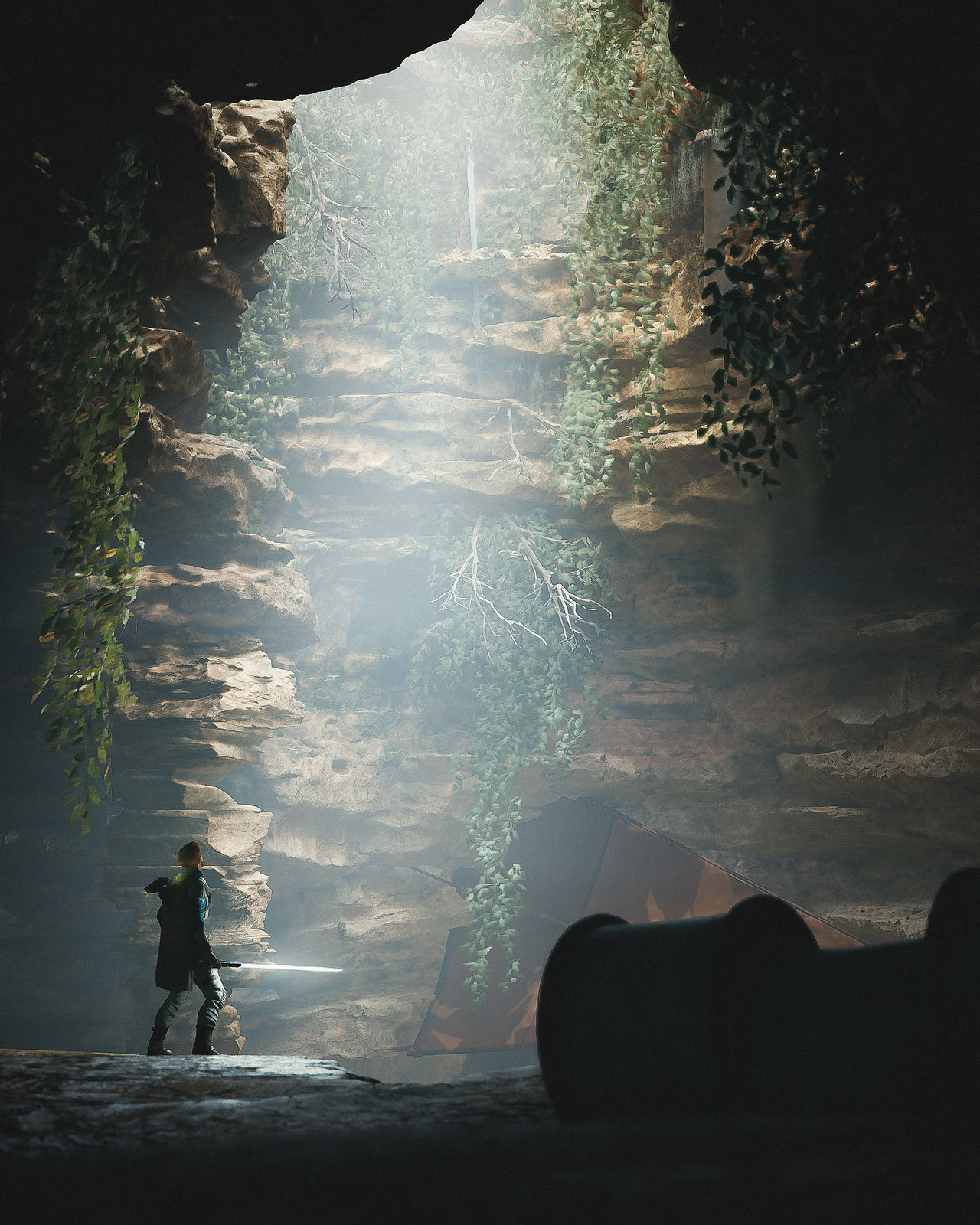A vertically rectangular image, likely computer-generated or a screenshot from a film, captures a dramatic scene in the lower left corner. A figure stands with legs apart, donned in a sweeping cape, their back facing the viewer. They gaze upwards towards the top of the frame, where a brilliant light penetrates the gloom of a vast cavern. The person's right hand wields an extended lightsaber, its blade glowing as it stretches horizontally towards the center of the frame. The cavern hosts an array of horizontal rock formations, adorned with trees and branches that grow downward, enhancing the otherworldly ambiance of the scene. The illumination from above casts an ethereal glow, highlighting the natural intricacies of the cavern.